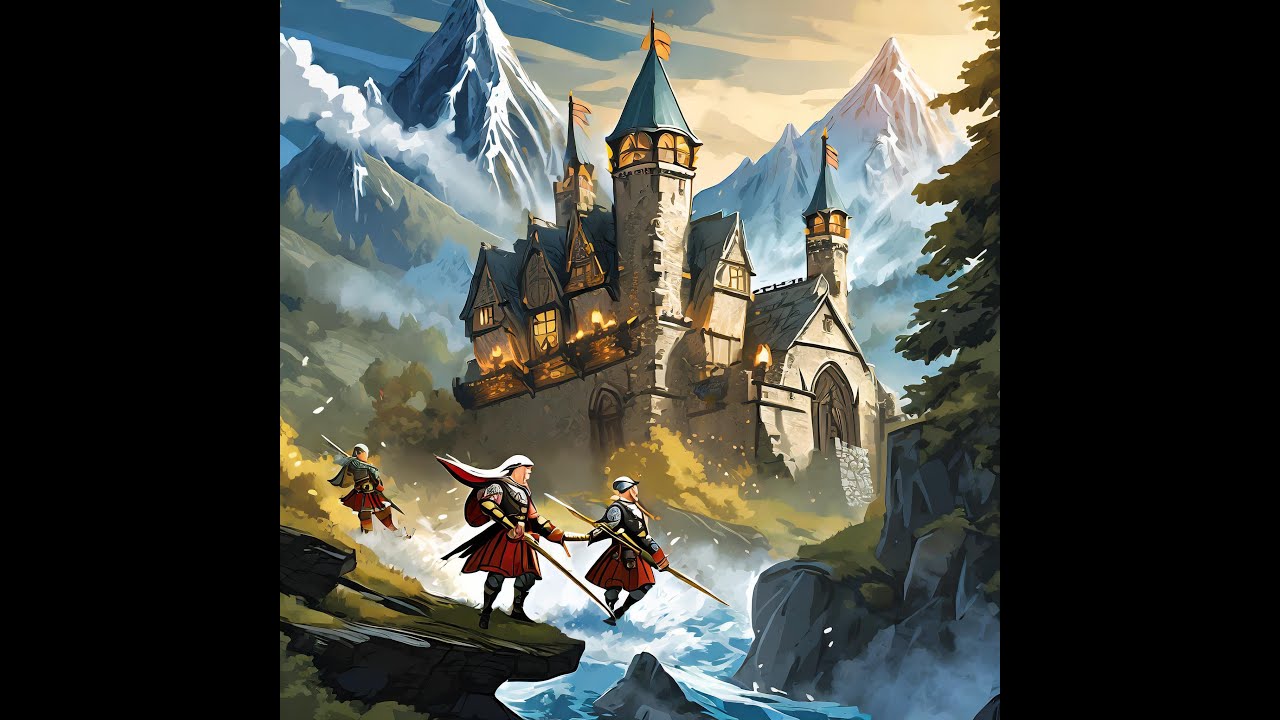This watercolor painting depicts a grand, medieval-style castle set against a backdrop of three towering, snow-capped mountain peaks. The castle, adorned with blue roof tiles and orange flags fluttering from its steeples, exudes a warm glow from its illuminated windows and fiery lanterns hanging outside. Its architecture features multiple triangular-shaped roofs and numerous windows, highlighting its grandeur. In the foreground, three soldiers dressed in red kilts, black armor, and helmets stand near a crystal blue river that could be part of a moat surrounding the castle. Each soldier is equipped with a spear and shield, evoking a Viking or Scottish appearance. A large green evergreen tree stands to the right of the image, next to some boulders, enhancing the scene's natural beauty. The overall setting suggests a fantasy world captured at sunset, with a blend of blue, white, and gray hues painting the mountains in the background.